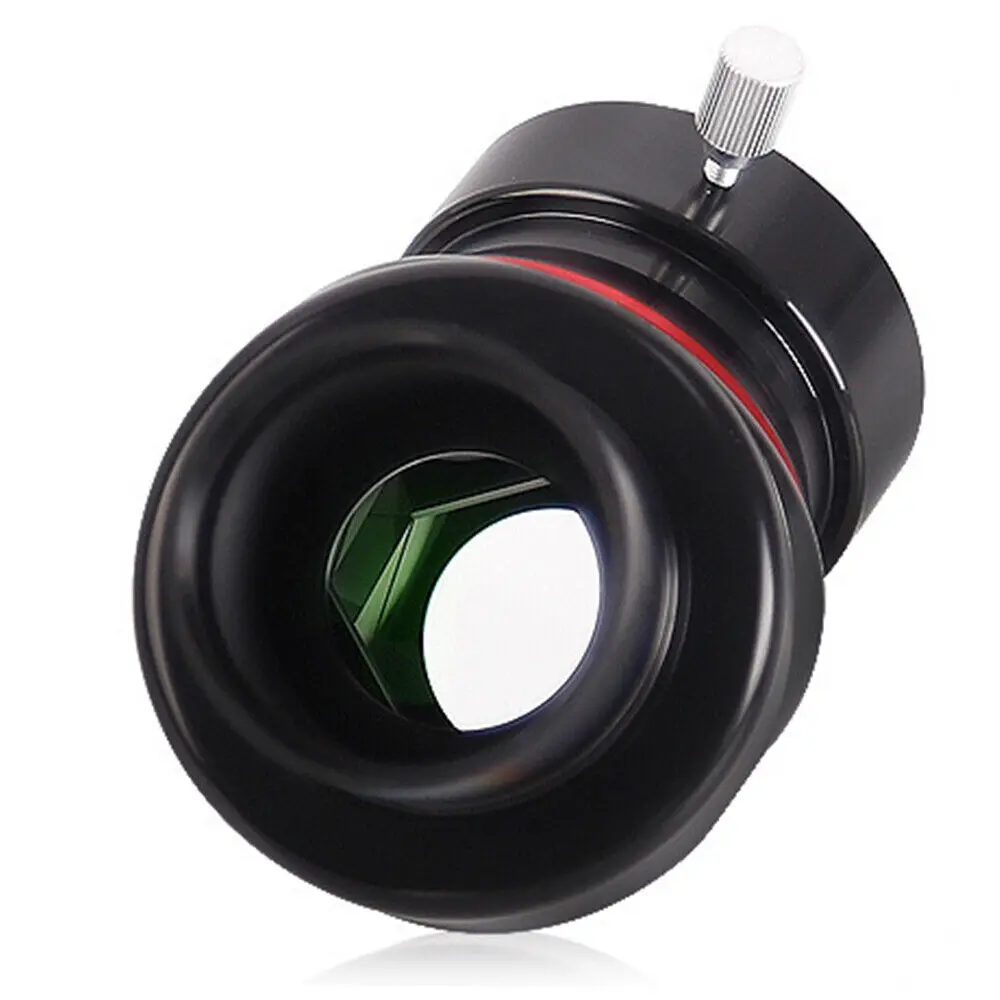This image features a mysterious black device with an ambiguous function, sitting against a white background. The device has a distinctive round shape with two circular ends, and a prominent silver metallic thumb screw or dial situated at the top, likely for attachment or adjustment purposes. Around the midsection of the device, there's a striking red ribbon-like border. The focal point is directed towards the silver knob and the red band. Inside one end of the device, you can see an opening that reveals a green internal component, possibly an aperture, suggesting it might have something to do with optics. The device is composed of materials that look like black plastic or metal, and it also features ridged detailing. While its precise function is unclear, the general consensus leans toward it being some form of lens or a fixture for a camera, projector, or plumbing system.